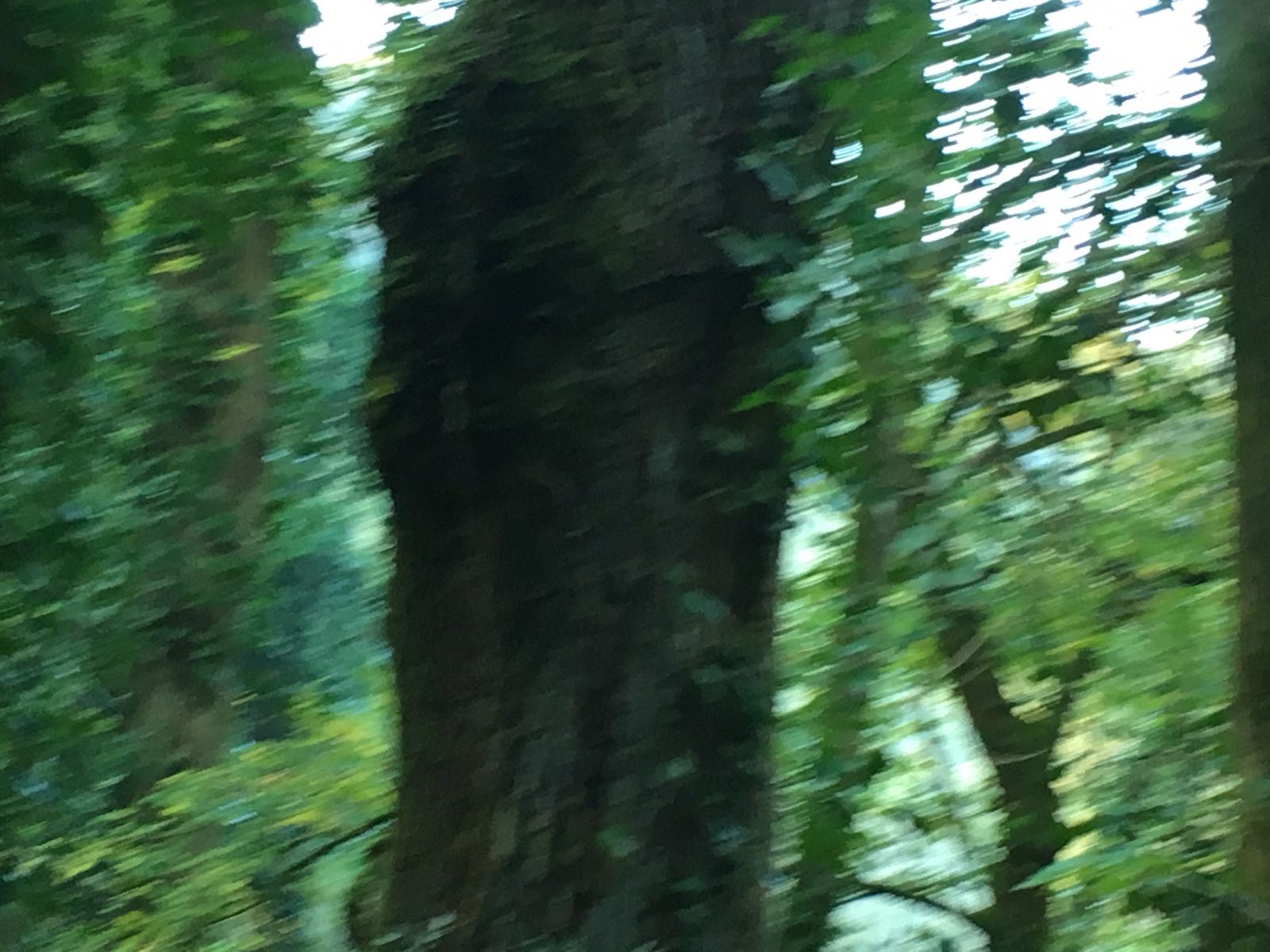A blurry and somewhat ambiguous image that could either be a photograph or an artwork, depicting an outdoor forest scene abundant with green foliage. Dominating the center is a prominent, dark tree trunk, almost black with varying shades of green interwoven throughout. This central tree creates a striking focal point amidst the verdant backdrop. Flanking the scene on the left, a dense cluster of trees, with only slight penetration of sunlight, adds to the lush ambiance. On the right side, a distinguishable tree extends its branches in a Y-shaped formation, adorned with leaves that spread out elegantly. Near the center stands another tall, slender tree, its height accentuated by a canopy of leaves, contributing to the layered depth of the woodland vista.